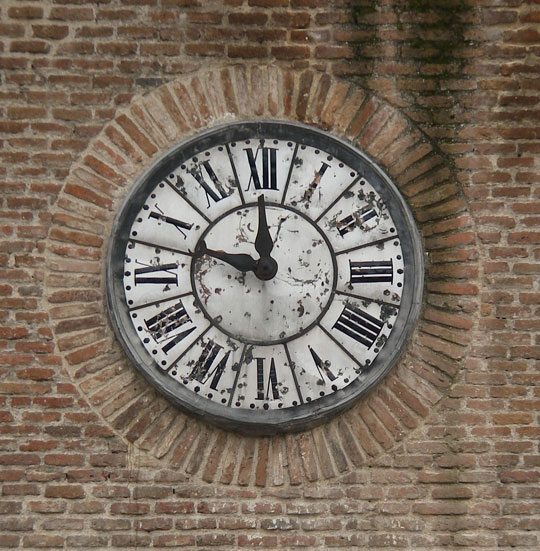This color photograph captures a vintage round clock embedded in a rustic stone wall composed of small red bricks. The bricks surrounding the clock are arranged in a radial pattern, creating a visually striking contrast to the horizontally placed bricks in the corners of the image. The clock features a grey-edged casing with a white face that appears aged or significantly dirty, indicating years of exposure or neglect. Roman numerals mark the hours, and thin lines separate each numeral. There is an inner circle at the center where the black clock hands meet. Both hands are almost identical in size, making it unclear whether the time shown is 10:00 or 11:50. The overall scene evokes a sense of timelessness and history, accentuated by the weathered appearance of the clock face.